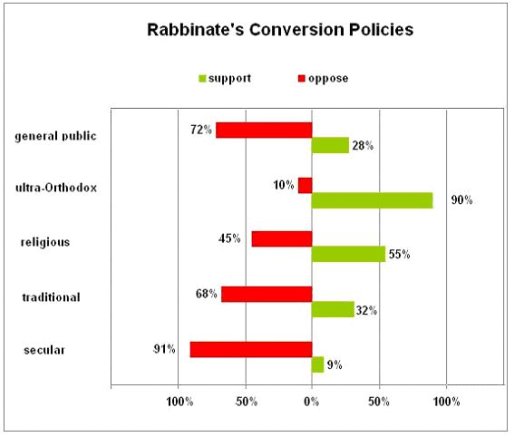The image is a detailed bar chart titled "Rabbinate's Conversion Policies" against a white background. The chart uses lime green bars to signify support and red bars to indicate opposition. On the left side of the chart, it categorizes responses from five distinct groups: General Public, Ultra-Orthodox, Religious, Traditional, and Secular. Each category has corresponding bars depicting the percentage of support and opposition. For the General Public, 72% oppose while 28% support. Among the Ultra-Orthodox, 10% oppose and 90% support. The Religious group shows 45% opposition and 55% support. Traditional respondents indicate 68% opposition and 32% support. Lastly, the Secular group has the highest opposition at 91%, with only 9% in support. Along the x-axis, the chart displays percentages ranging from 0% to 100% for both support and oppose, providing a clear visual comparison across different societal segments.